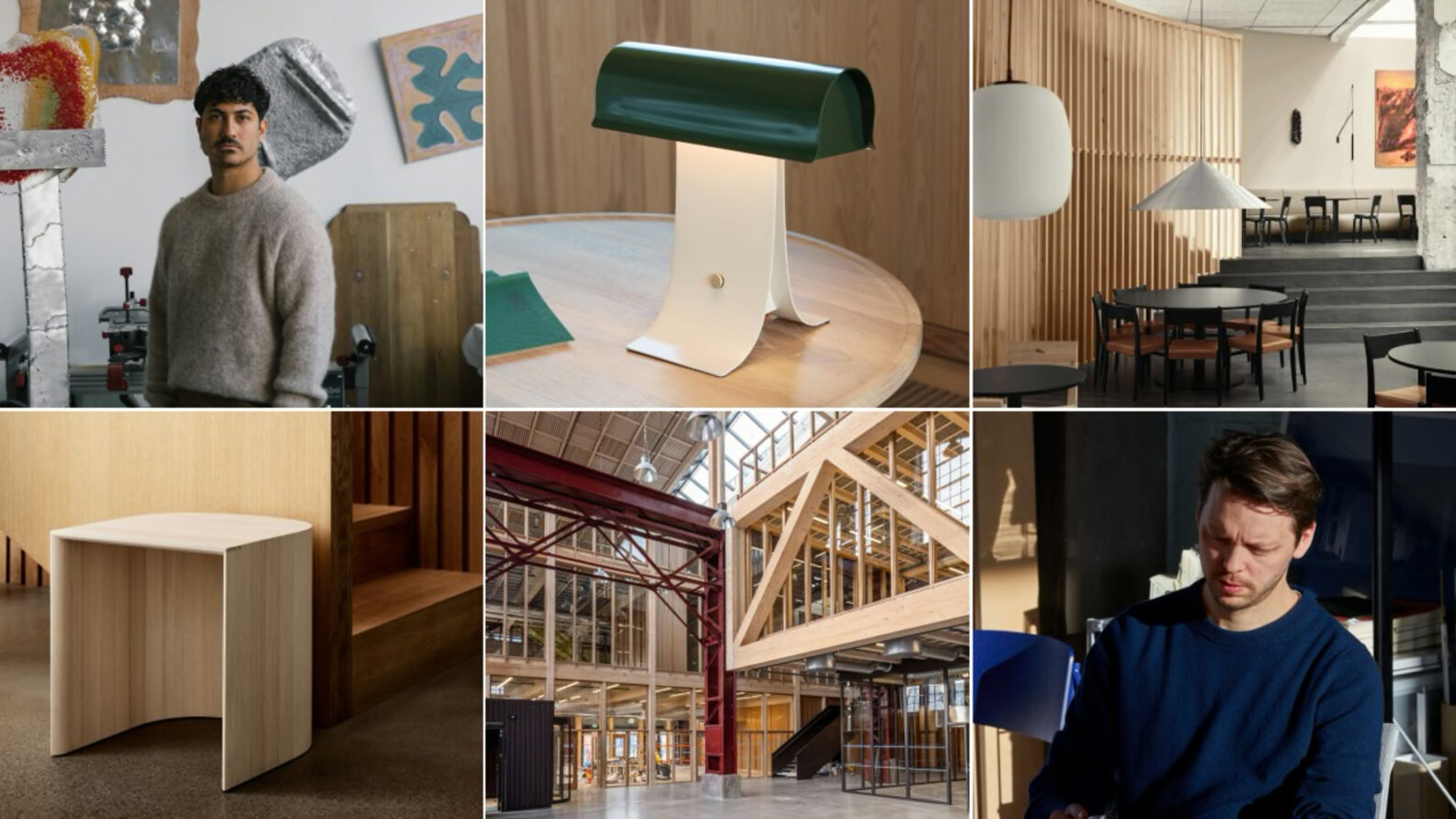The image is a collage consisting of six square photographs arranged in two rows. The top row features, from left to right: a young man in a gray sweater standing before a backdrop adorned with various artworks; an industrially designed lamp with a white, rectangular base that curves into a straight line supporting a half-rounded, green cylindrical lampshade; and a stylish dining area with black tables, some topped with modern hanging lamps, including a white oval one and a half-triangular shaded one. The bottom row, again from left to right, includes: a plain, unfinished plywood chair with a curved back and open center; an interior view of a building with bare plywood framing for windows, structures, and pillars; and finally, a white male with wavy blonde hair dressed in a blue sweatshirt. Each image portrays a unique element of modern design and architecture.